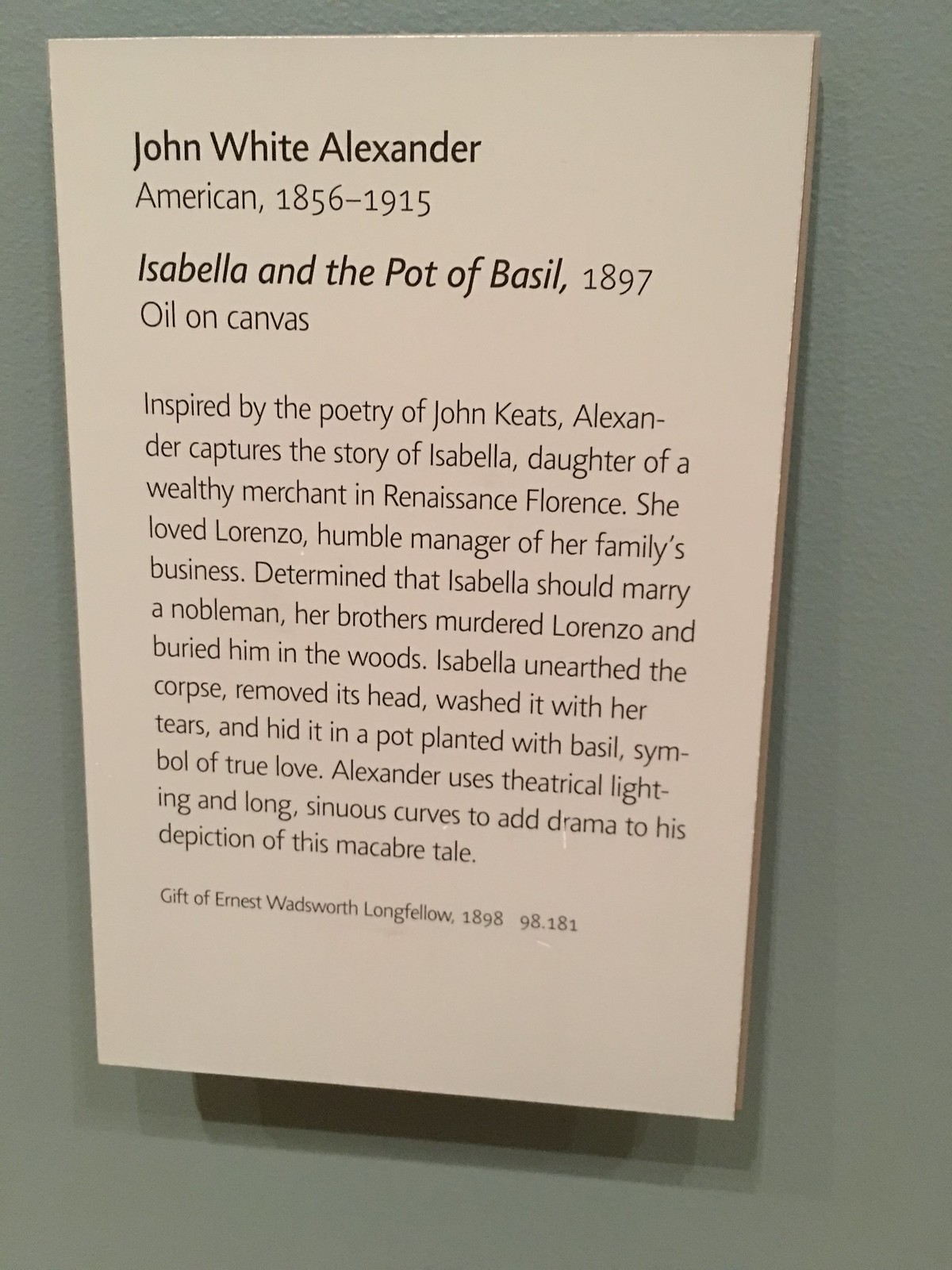This detailed descriptive caption combines key elements from the three provided captions, highlighting shared and repeated information while enhancing it with a cohesive narrative:

---

This is a photo of a placard describing an artwork created by American artist John White Alexander (1856-1915). The placard, tan in color, hangs on a gray wall, likely within a museum. At the top, in uppercase black letters, it reads: "John White Alexander, American, 1856-1915." Below this, in bold font, it states the title "Isabella and the Pot of Basil, 1897," specifying it as an oil painting on canvas. This piece was inspired by the poetry of John Keats and tells the haunting story of Isabella, a daughter of a wealthy merchant in Renaissance Florence. Isabella fell in love with Lorenzo, a humble manager in her family's business—a liaison her brothers disapproved of. Determined that Isabella should marry a nobleman, they murdered Lorenzo and buried his body in the woods. Isabella subsequently unearthed Lorenzo's corpse, removed his head, and, after washing it with her tears, concealed it in a pot planted with basil, symbolizing true love. John White Alexander's rendition of this macabre tale employs theatrical lighting and elongated curves to heighten the drama and emotion of the scene. This painting was a gift from Ernest Wadsworth Longfellow in 1898, cataloged as 98.181.

---